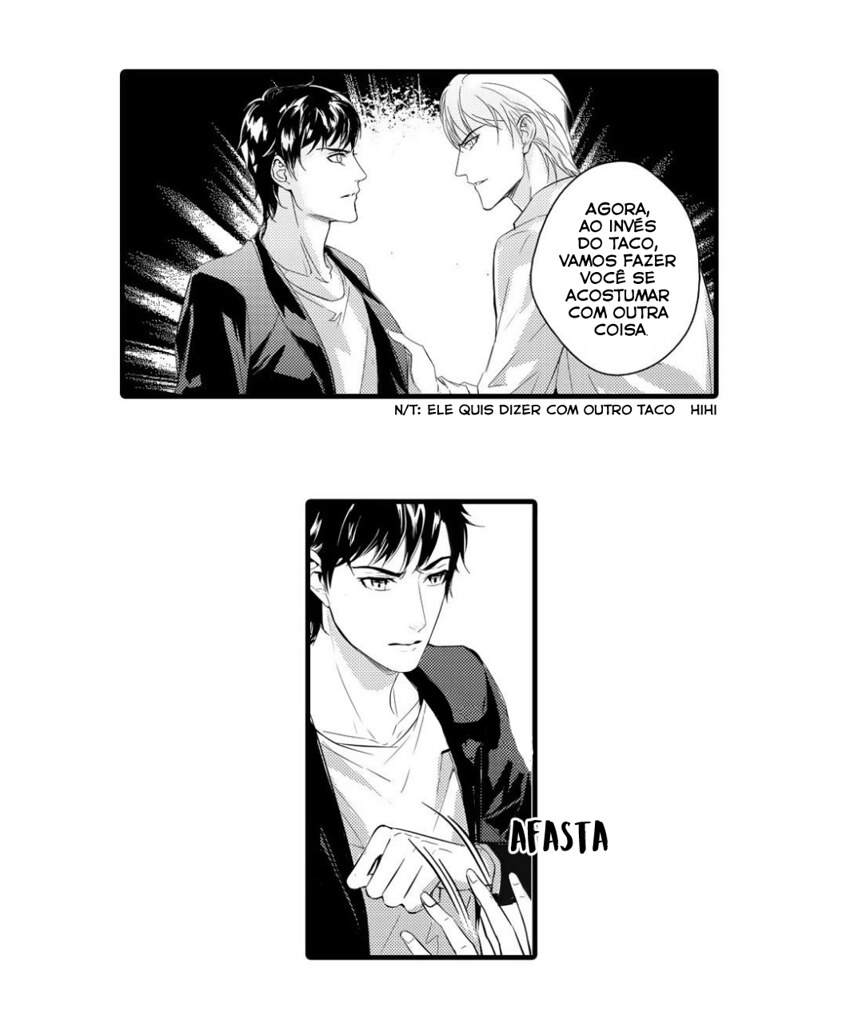The image consists of two black-and-white cells from a graphic novel styled as a Japanese manga, with text seemingly in Portuguese. 

In the upper cell, which is a horizontally long rectangle, two young men face each other in profile, appearing to confront one another. The man on the left has black hair and wears a black jacket, while the man on the right has white or blonde hair and wears a white jacket. They are engaged in a tense moment, with the white-haired man grabbing the lapel of the black-haired man's jacket. The text in the speech bubbles reads, "Agora eu inves do taco, vamos fazer você se acostumar com outra coisa," suggesting a heated conversation. 

The lower cell focuses solely on the black-haired man, who is now shown pushing the white-haired man's hand away. This frame is narrower and captures the black-haired man's upper torso and head, facing forward. His left hand is raised to his chest as he shoves the other's hand aside, with the word "Afasta" prominently overlaying the image, indicating the action of pushing away.